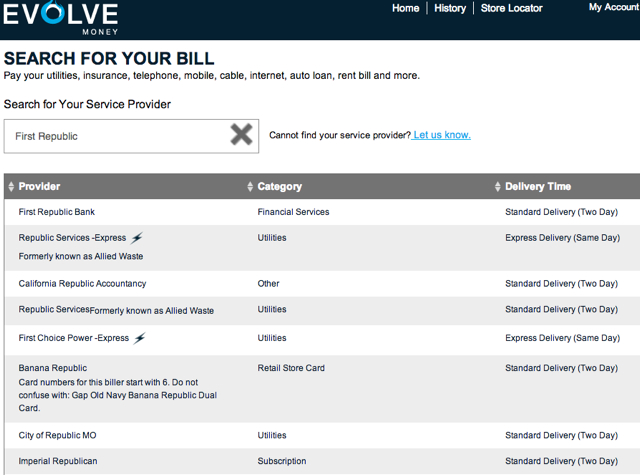This image is a screenshot of an application called Evolve Money. At the top of the interface, there's a black menu bar featuring the Evolve Money logo on the upper left-hand side. On the right-hand side of this bar, there are several navigation options: Home, History, Store Locator, and My Account. Below the menu bar, against a white background, bold black text reads "SEARCH FOR YOUR BILL" in all capital letters. Underneath, it states "Pay Your Utilities, Insurance, Telephone, Mobile, Cable, Internet, Auto Loan, Rent, Bill, and More."

Further down, the text "Search for Your Service Provider" is shown above a search bar that includes the pre-filled text "First Republic" and a large gray 'X' at the end of the search box for clearing the input. Adjacent to the search bar is a prompt reading "Cannot Find Your Service Provider?" accompanied by a clickable blue text link stating "Let Us Know."

The lower part of the image displays eight service listings against alternating white and gray backgrounds. These listings are categorized under the headers: Provider, Category, and Delivery Time. The listed service providers include:

1. First Republic Bank
2. Republic Services Express
3. California Republic Accountancy
4. First Choice Power Express
5. City of Republic, Missouri
6. Imperial Republican

Each provider entry is presented with corresponding details pertaining to its category and estimated delivery time.